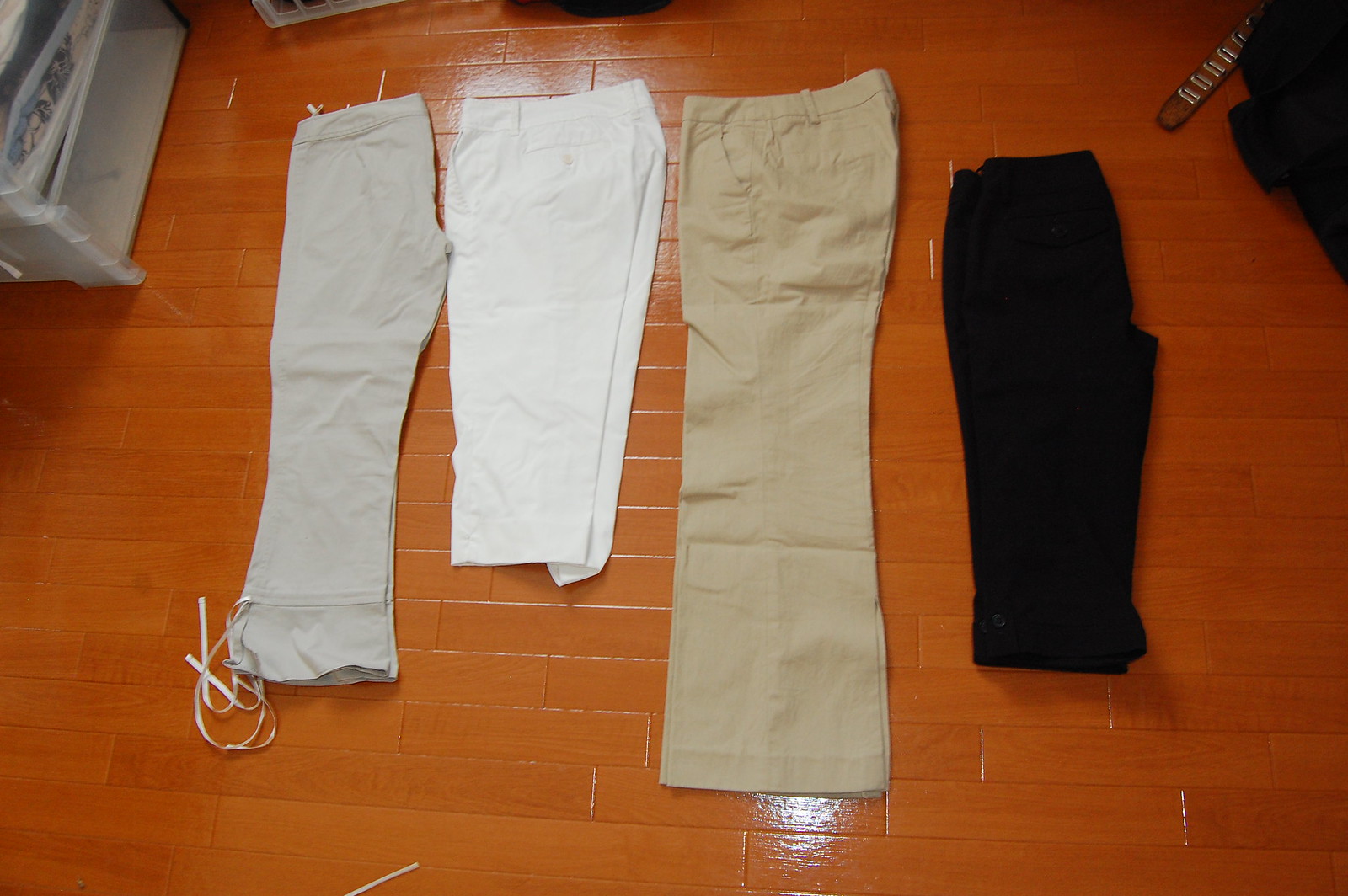The photograph showcases a collection of four pairs of pants neatly laid out on a wooden floor painted in a reddish-sienna hue. The floor features a wood grain pattern with a slight shine, reminiscent of polished wood or possibly even brick. The pants are arranged side-by-side, each folded in half lengthwise, displaying their full length. From left to right, the lineup includes a pair of black pants, a beige pair, a short white pair resembling capris, and green pants with ties at the bottom cuffs, possibly for adjusting the fit similar to sweatpants. To the right of the pants, there's additional dark clothing and a belt. In the background, shelves can be seen, suggesting the setting might be a store where these new pants await folding and display.